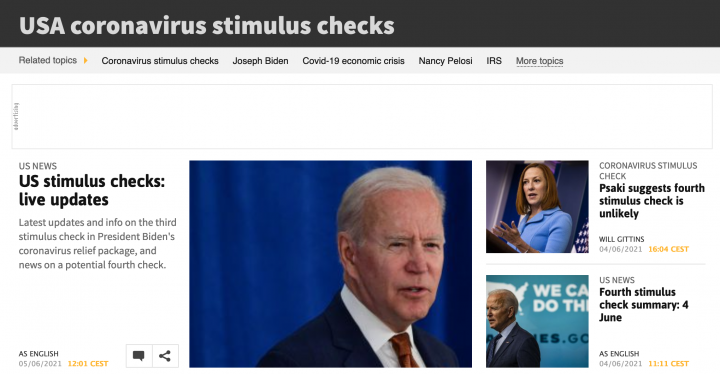The image depicts a low-quality news website focused on U.S. national news, predominantly addressing the topic of Coronavirus Stimulus Checks. The top portion features a prominent headline that reads "USA Coronavirus Stimulus Checks" followed by related topics such as Stimulus Checks, Joseph Biden, COVID-19 Economic Crisis, Nancy Pelosi, and IRS. The main content area includes three primary articles about the U.S. Stimulus Checks, with titles like "Live Updates."

On the right-hand sidebar, there is an article about Jen Psaki, the former White House Press Secretary, titled "Psaki Suggests Fourth Stimulus Check is Unlikely," alongside another article related to the Fourth Stimulus Check. The site is cluttered with a slew of articles generated by AI, focusing on trending topics to drive clicks, hinting at its lack of reliability and quality.

Visually, the site is dominated by a stark white background with sporadic black text. There are two images of Joseph Biden and one of Jen Psaki, emphasizing the political figures associated with the stimulus checks. The overall aesthetic of the site appears unprofessional and untrustworthy, catering to individuals hoping for additional stimulus checks amidst the economic crisis triggered by COVID-19.